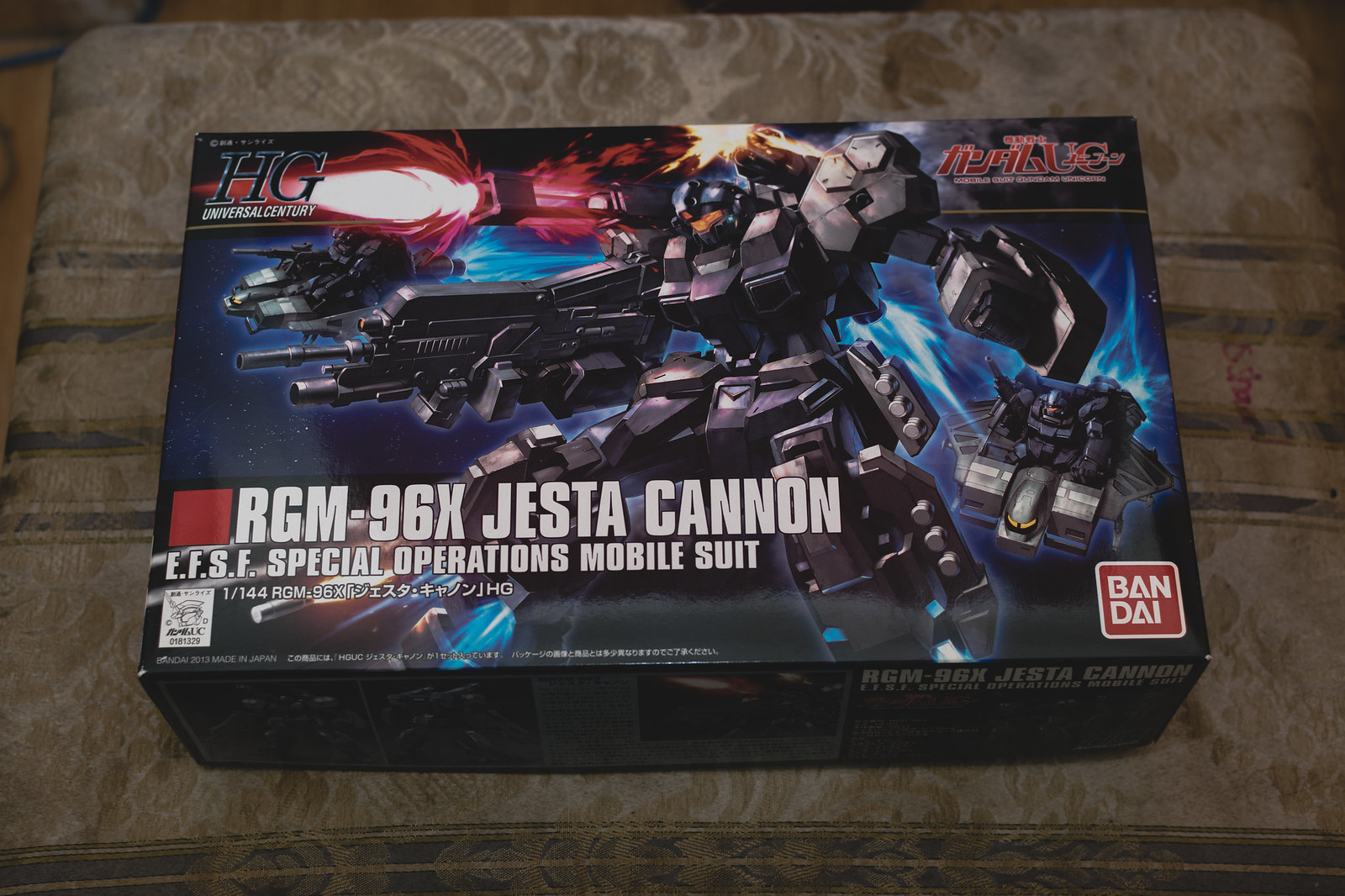The image is a detailed photograph of a box featuring a highly detailed action figure or model kit. The box, labeled "RGM-96X Jesta Cannon EFSF Special Operations Mobile Suit," sits atop a brown seat or footstool, possibly made of aged fabric. The box itself is primarily black, adorned with an intricate graphical depiction of the Jesta Cannon mobile suit, which appears partly robotic with elaborate weaponry, including guns and cannons. The illustration on the box suggests dynamic motion, possibly with the mobile suit firing its weapons. 

In the top left corner, the text "HG Universal Century" is prominently displayed, while the top right corner contains Japanese characters in red font. The bottom right corner features the Bandai logo in a white font on a red background with a white border. The bottom left corner also has a red square with white text, identifying the model explicitly: "RGM-96X Jesta Cannon" followed by "EFSF Special Operations Mobile Suit" in smaller text. Additional logos and Japanese letterings are scattered around the upper sections of the box, merging Eastern and Western branding. The box is a product of Bandai, a well-known Japanese manufacturer, emphasizing its authenticity and origin.